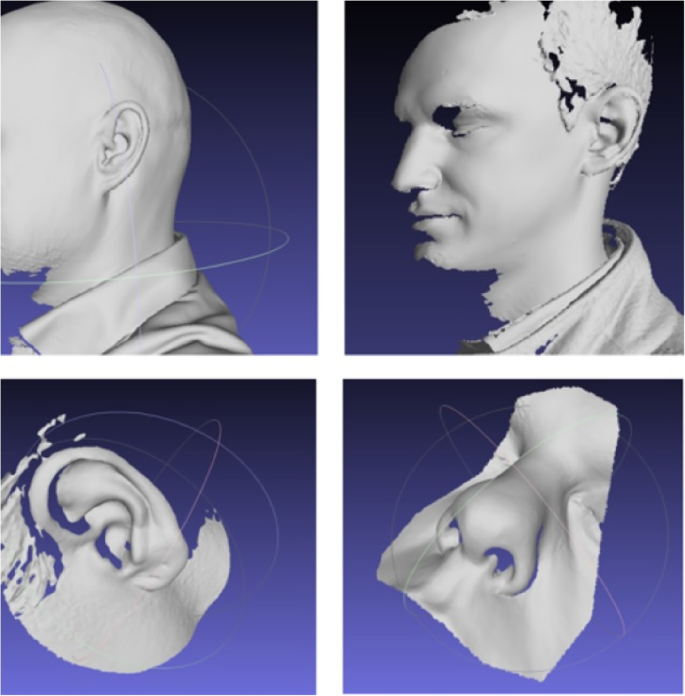The image is a vertically rectangular digital piece divided into four distinct sections by white borders. Each section contains a 3D monochromatic sculpture of different parts of a man's face, set against a dark purple background. The upper left corner showcases a side view of the man's bald head, visible from just behind the eyes and nose to the back of the head. In the upper right, the same man is depicted in profile with a laurel-like crown, showing his closed eye, nose, and mouth. The bottom left features a close-up of an ear, while the bottom right displays a detailed view of the man's nose and eye sockets. The image is well-lit and each section is clear and detailed, emphasizing the sculptural quality of the facial features.